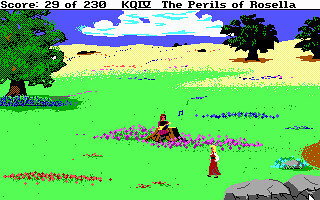In this highly pixelated, nostalgic 8-bit video game scene from "KQIV: The Perils of Rosella," the screen displays "Score 29 of 230" at the top in black text. The vibrant landscape features a green lawn adorned with clusters of colorful flowers—blue, pink, and red. A prominent rounded tree with green leaves and brown trunk stands on the left, and two smaller trees are positioned in a sandy brown area further back. Two gray rocks lie in the bottom right corner.

The backdrop reveals a mesmerizing purple sky streaked with hues of blue, accompanied by a large, billowy white cloud. In the midst of the scenery, a figure wearing red pants, a white shirt, and brown hair sits on a tree stump, playing a musical instrument, with a blue musical note hovering above. Towards the musician, a blonde-haired woman in a brown dress appears to be walking, possibly dancing, adding a sense of movement and interaction to the serene environment. The entire scene echoes the charm of vintage video games, capturing a moment of simple yet captivating adventure.